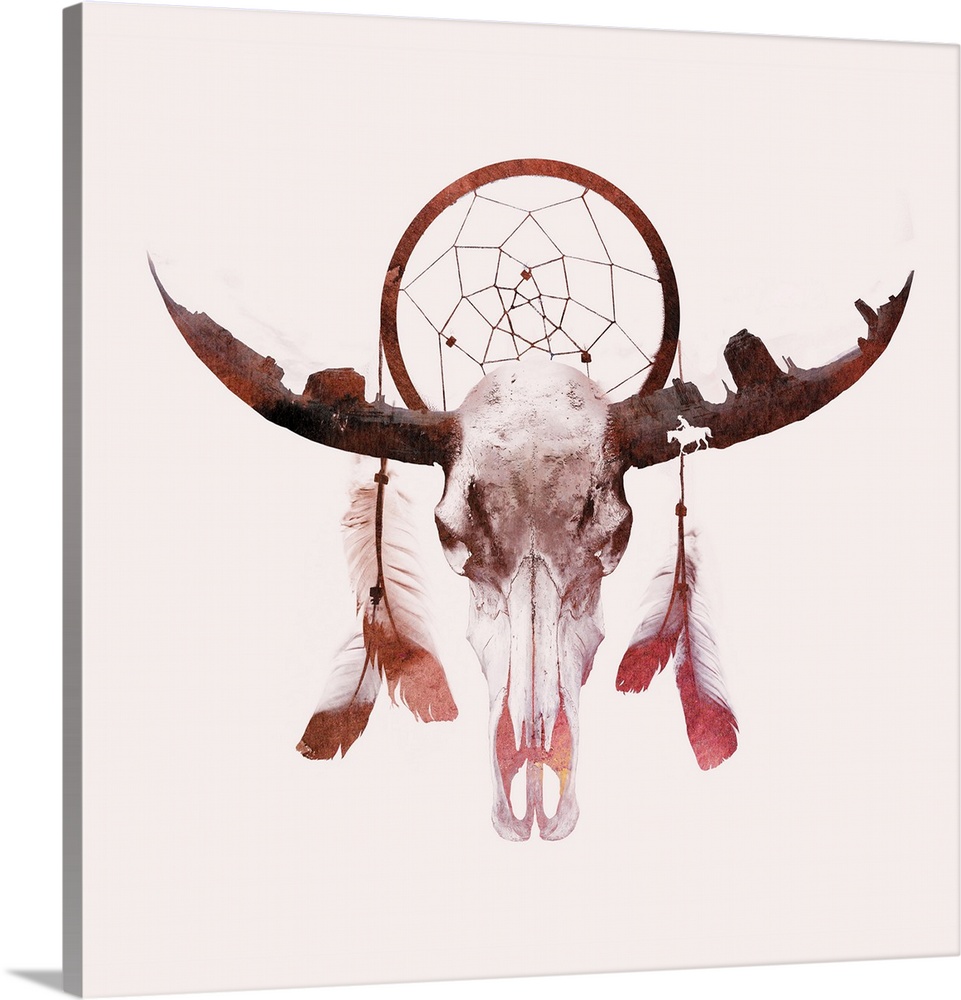The image depicts an art piece set against an off-white canvas background, subtly shadowed on the left to show dimension. At the center, a buffalo skull features prominently, its irregular and ragged horns pointing upward. Uniquely, the skull's head is transformed into a dreamcatcher, a circular object with a cobweb-like string pattern inside. Adorning this dreamcatcher are two sets of ribbons with beads, hanging elegantly. Feathers, mostly white with touches of orange-red at their tips, dangle from the horns. The horns themselves, short and pointed, subtly resemble a desert mesa landscape. To the right, a tiny silhouette of a man on a horse completes the composition, adding a sense of narrative and depth to the scenery. The piece employs a palette of rust red, white, and brown, blending harmoniously to evoke a sense of the vast, rugged desert.